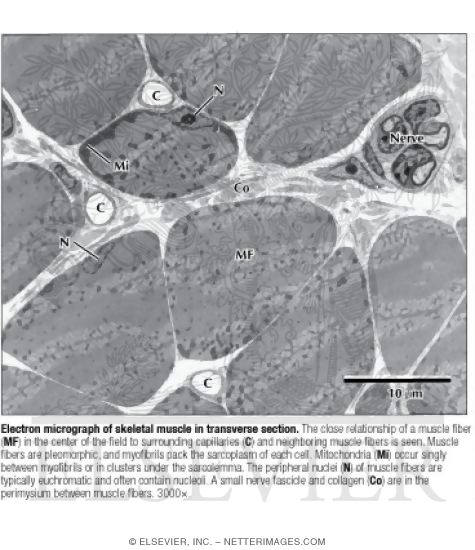This black-and-white image is a detailed electron micrograph of skeletal muscle in transverse section. Dominated by swirling patterns of white, gray, and black, it presents an intricate view reminiscent of something observed under a microscope. Key elements are labeled meticulously: the muscle fibers as MF, the capillaries as C, mitochondria as MI, nuclei as N, collagen as CO, and the nerve simply labeled as 'nerve'. A grainy legend in the corner indicates that each line represents 10 micrometers. The photo reveals the close relationship of a muscle fiber at the center to its surrounding capillaries and includes several intricate web-like connections between nerves and the muscle itself. This scientific image, possibly derived from a textbook or medical research paper, is further explained by a description at the bottom that reads: "electron micrograph of skeletal muscle in transverse section," with additional explanatory text about the muscle structure and associated components.